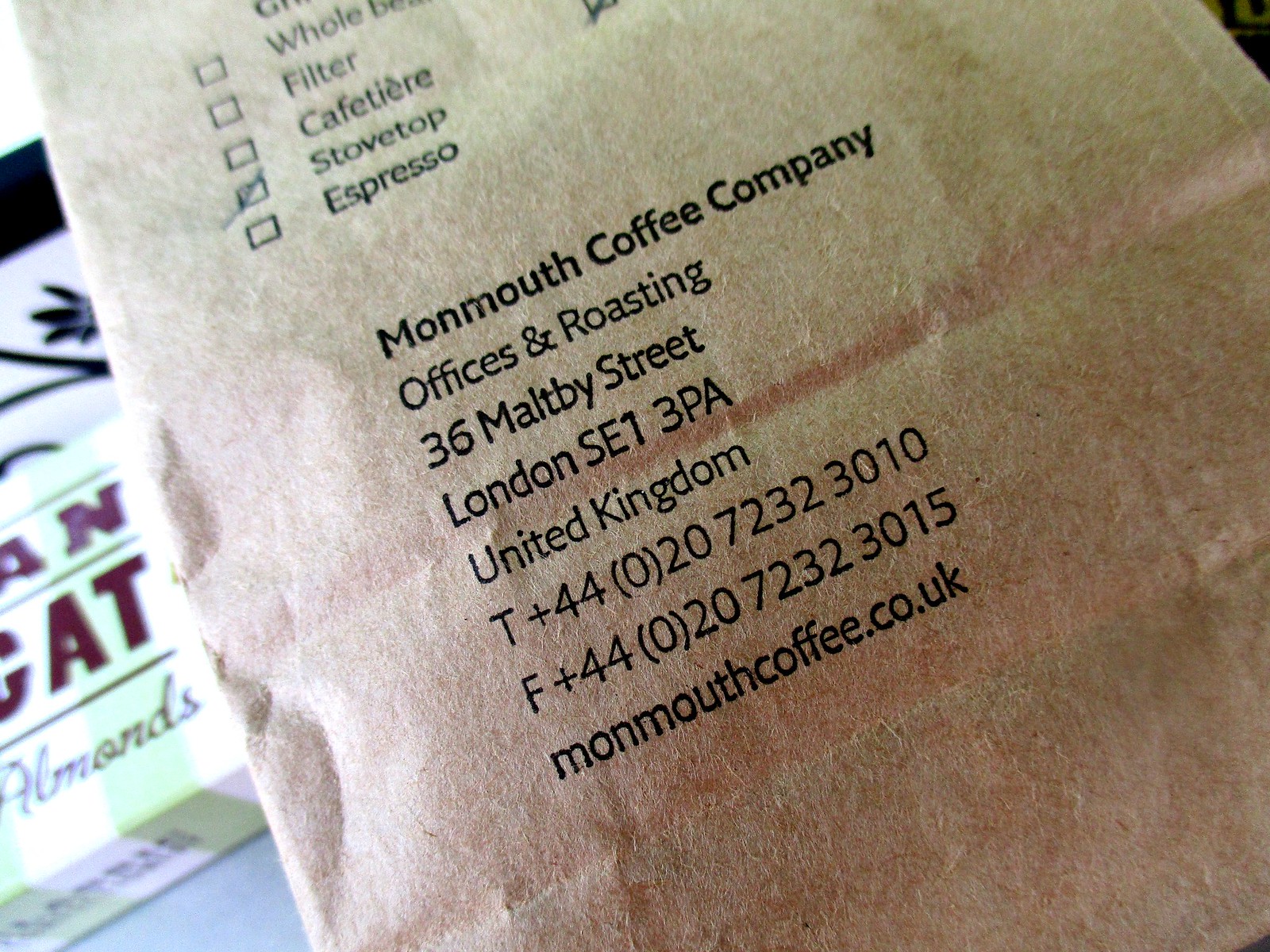This is a detailed close-up photograph of an order receipt for Monmouth Coffee Company, printed on what appears to be a brown paper bag. At the top of the receipt, various coffee preparation categories are listed: Whole Bean, Filter, Cafetray, and Stovetop, with the Stovetop box marked with a check. Below this section, the company’s details are prominently displayed in black text: Monmouth Coffee Company, Offices and Roasting, 36 Maltby Street, London, SE1 3PA, United Kingdom, along with telephone numbers and the website address, monmouthcoffee.co.uk. The brown paper bag is situated atop some other boxes, with one visible at the bottom left corner labeled "Almonds," which is white with green stripes.